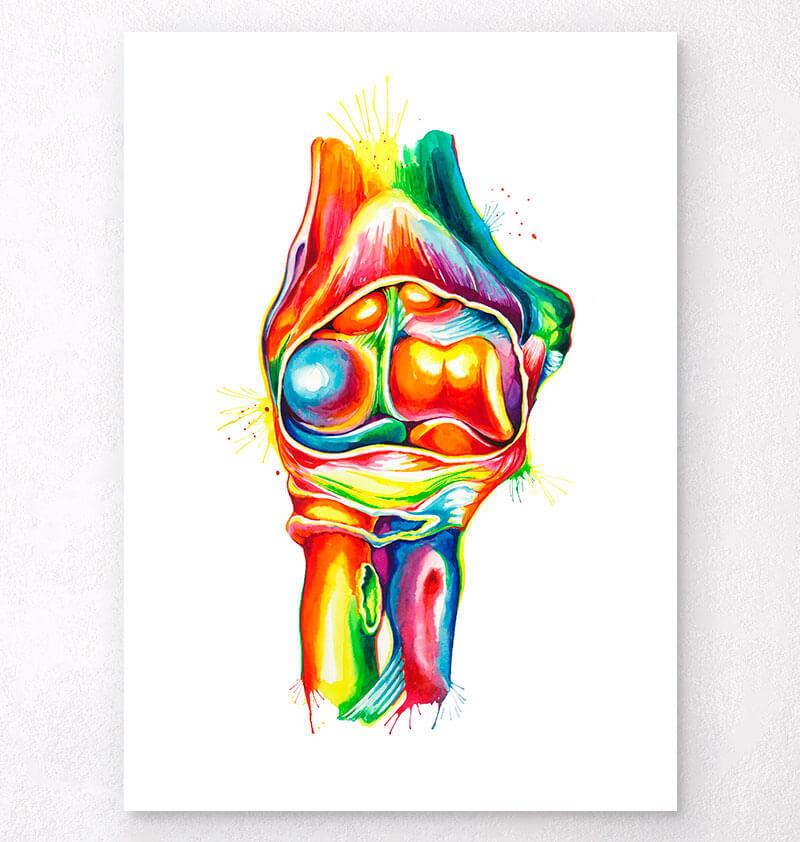This vibrant watercolor painting, executed in a dazzling array of saturated neon hues—featuring yellows, oranges, hot pinks, purples, teals, and blues—depicts an organic, anatomical structure reminiscent of a knee joint without skin, showcasing intricate details with parts of cartilage and bone. The composition, which might suggest a slightly surreal or animalistic interpretation due to additional elements, skillfully integrates rounded and tubular forms that come together in a crisp, clear manner. The artwork is mounted on a stark white canvas with a slightly textured background, enhancing its vivid, un-gory appearance and making it stand out brilliantly.